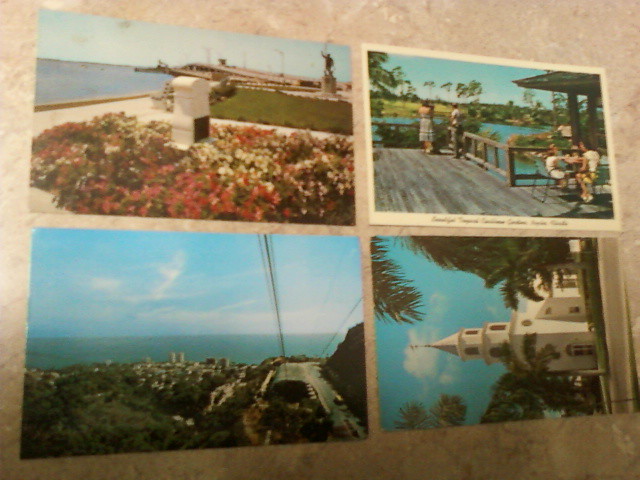An image showcases four picture postcards laid out on a surface resembling concrete or a concrete-esque island table. These postcards depict various travel destinations, each offering a glimpse into unique sceneries. 

The top left postcard features a picturesque scene with a bed of red and white flowers in the foreground, accompanied by what appears to be a stone monument. Beyond this, a bronze statue on a pedestal overlooks a tranquil waterway, with a long causeway or overpass bridge stretching out in the distance. This scene hints at a serene blending of nature and man-made beauty.

To the right, the second postcard illustrates a tropical escape. It pictures a wooden deck overlooking vibrant blue waters. On the deck, two individuals gaze out at the horizon, surrounded by palm trees swaying gently in the background. There's also another figure seated at a table in the foreground, adding a sense of relaxed human presence to the idyllic setting.

The third postcard, located at the bottom right, offers a panoramic view that appears to be from a gondola or cable car, presenting an aerial perspective of a city and its adjoining bay. The vista resembles a dramatic scene from Gibraltar, showcasing the city stretching below, the expansive ocean, and the sunlit sky on the horizon.

Lastly, the fourth postcard portrays a white chapel with an elegant steeple reaching into a clear blue sky. The church is bordered by green foliage, possibly palm trees, which add a picturesque and tranquil charm to the sacred structure.

Together, these postcards create a rich tapestry of diverse landscapes, capturing monuments, tropical retreats, coastal vistas, and serene chapels, each telling its own story of the destinations visited.